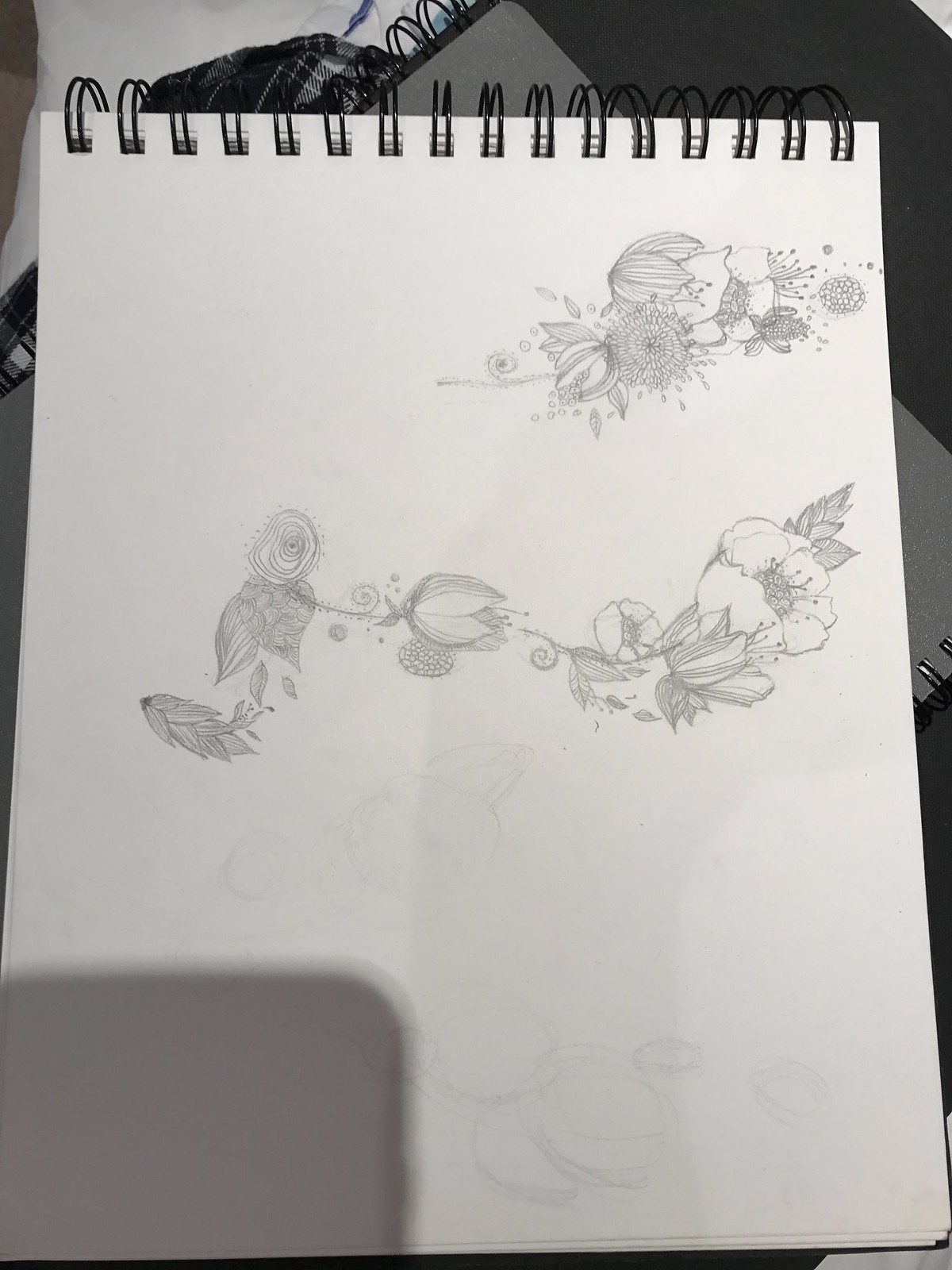This portrait-oriented photograph captures an intricate sketch on a white sketch pad with black ring-like binding at the top, enabling pages to be flipped over. The paper is stark white and contrasts sharply with the detailed artwork. In the bottom left-hand corner of the sketch pad, there is a solid gray rectangle. The top of the sketch pad features a delicate and diverse array of flowers, rendered with fine and meticulous detail that makes identification challenging from a distance. Just below this, roughly across the center of the page, there is another cluster of flowers, including a visibly closed rose. The entire sketch is executed in black and white, emphasizing the elegant and intricate designs of the floral subjects.